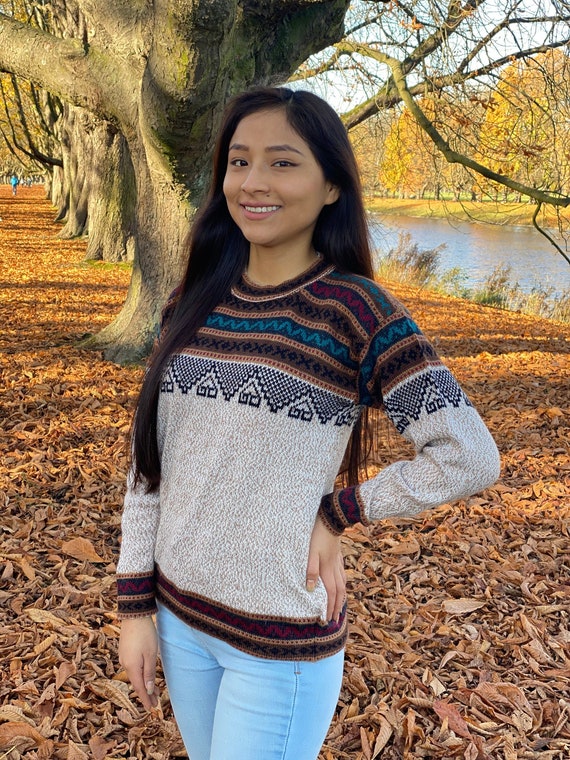In a picturesque autumn scene with a backdrop of golden and brown leaves, an Asian girl with long, dark hair smiles radiantly as she poses for the camera. Dressed in light blue jeans, she wears a distinctive knitted sweater that features intricate indigenous-inspired patterns in indigo, brown, tan, and hints of red across the top of the chest and sleeves. The main body of the sweater is a blend of beige and white, creating a static-like texture, and is accentuated by black geometric designs around the neck, sleeves, and waist. Her hand rests confidently on her hip, showcasing her sweater. Behind her, a tranquil river flows alongside a line of autumn-hued trees, and a faint figure can be seen in the distance past the tree line. A serene park setting with a pond further enhances the fall atmosphere, making the scene both vibrant and serene.